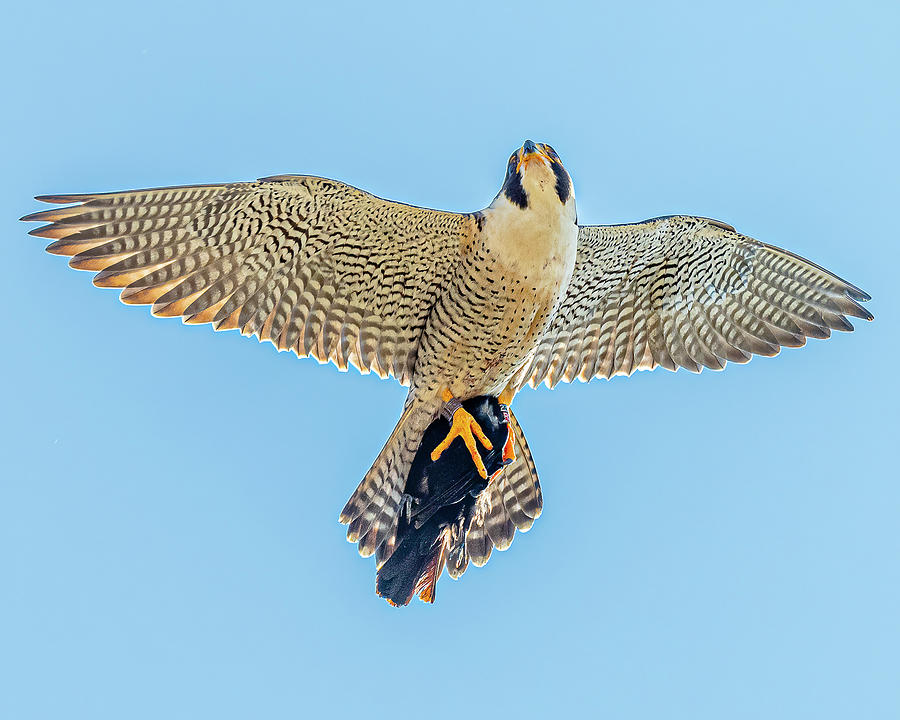The photograph captures a striking scene of a large bird of prey in flight against a watercolor blue sky. The bird, identified as a type of hawk, showcases an impressive wingspan with feathers that display a beautiful blend of blue, gray, and gold, possibly enhanced by the sunlight. Notably, its chest is white, with a blue streak running down both cheeks and part of its head also tinged blue. The hawk’s eyes are marked with black, and its beak is yellow with a black tip. The underbody and undersides of its wings feature a patterned mix of white and gray stripes. In its sharp yellow claws, the hawk clutches a smaller black bird, highlighting its predatory nature. Additionally, the hawk has a gray band around one leg, suggesting it may have been banded for research or could be a trained bird. This magnificent hawk, powerful and graceful in motion, provides a remarkable glimpse into the life of a raptor.